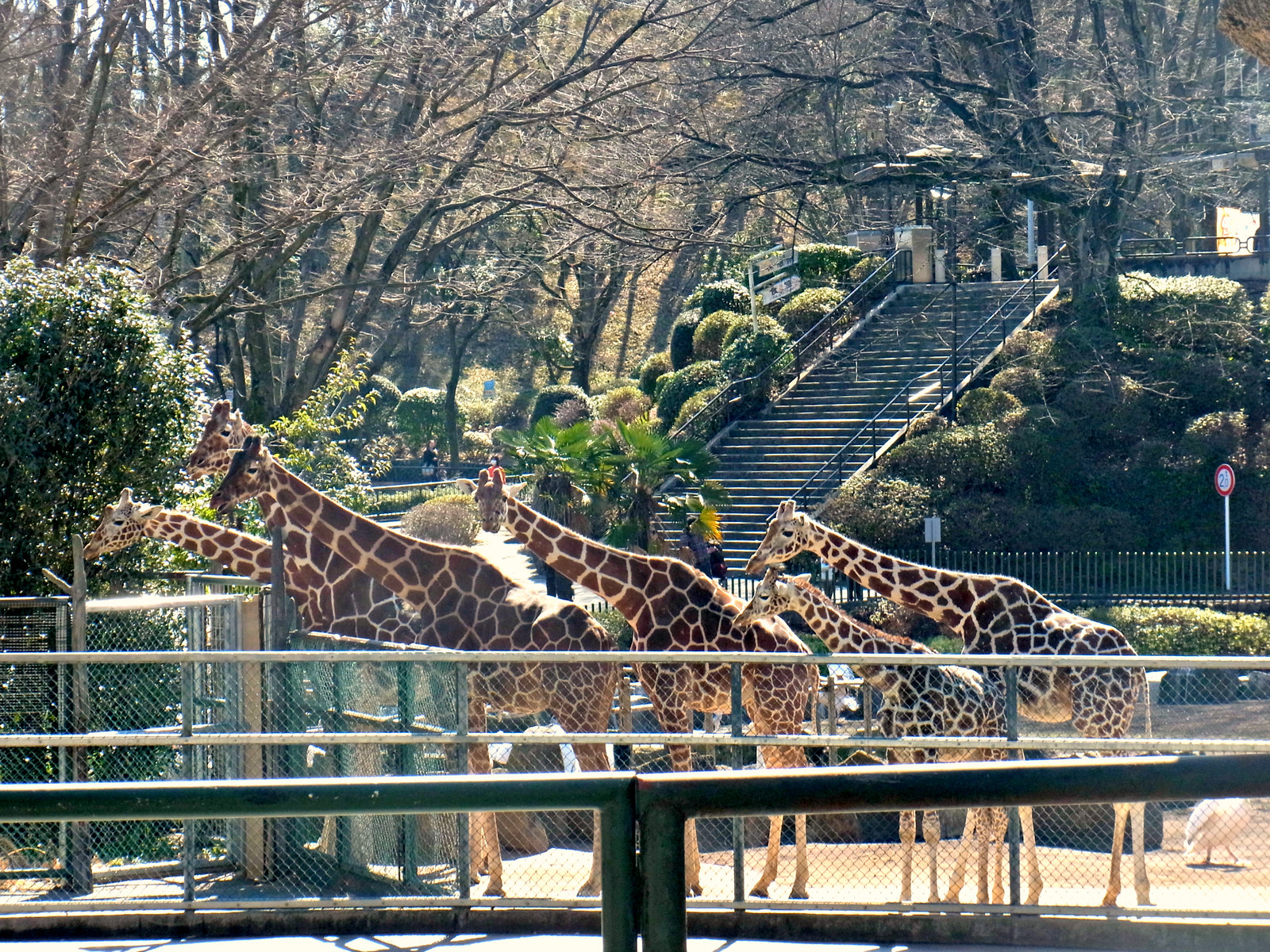This photograph captures a bright, sunny day at a city zoo, showcasing six giraffes of varying sizes within their enclosure. The giraffes, consisting of four adults and two juveniles, are lined up from left to right, gazing to the left side of the image as if waiting attentively. They stand behind a four-foot chicken wire fence, reinforced by an additional gate, creating a secure boundary between them and the visitors. A steep staircase with many steps descends in the background, partially surrounded by a mix of large, leafless trees and dense bushes, indicating a fall or winter setting. Adding to the scene, a white bird with visible wings is noticeable in the lower right corner of the image. The combination of natural and artificial elements, including the fenced enclosure and strategically placed road sign, seamlessly integrates with the zoo's wooded landscape.